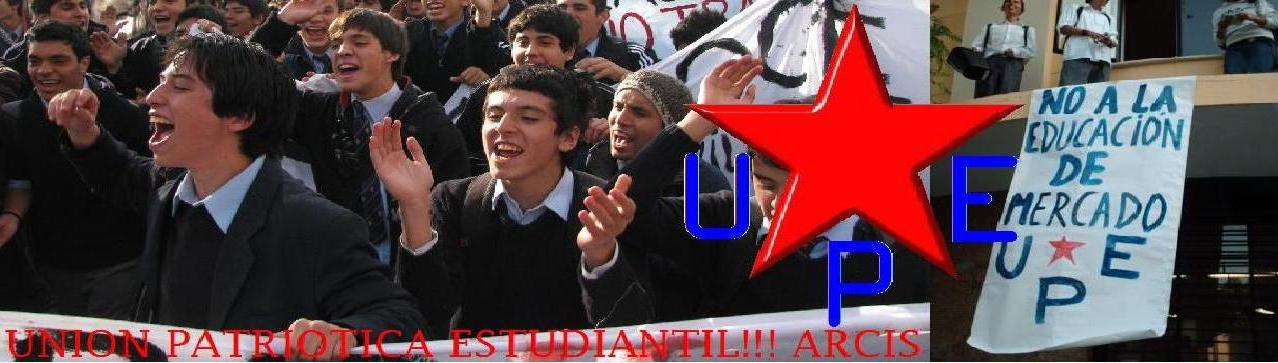The photograph, set outdoors during the day, features a lively group of primarily young Hispanic men, possibly at a rally or demonstration. They are uniformly dressed in dark sweaters or jackets paired with white or light blue button-down shirts, suggesting they might be in school uniforms. Notably, one of the young men is clapping his hands enthusiastically. Amongst the crowd, one man stands out by wearing a tie, and behind them, a woman in a grey cap is seen yelling. In the background, several students in white shirts and grey slacks watch from a balcony. The image is overlain by a graphic of a large red star with the letters UPE in purple between the star's points. Multiple signs and banners can be seen in the scene, including a prominent one that reads "No a la educación de mercado UPE." Additional signage with both black and red lettering is visible, though less legible. At the bottom of the photograph, red lettering spells out "Unión Patriótica Estudiantil ARCIS," reinforcing the collective and spirited nature of the gathering.